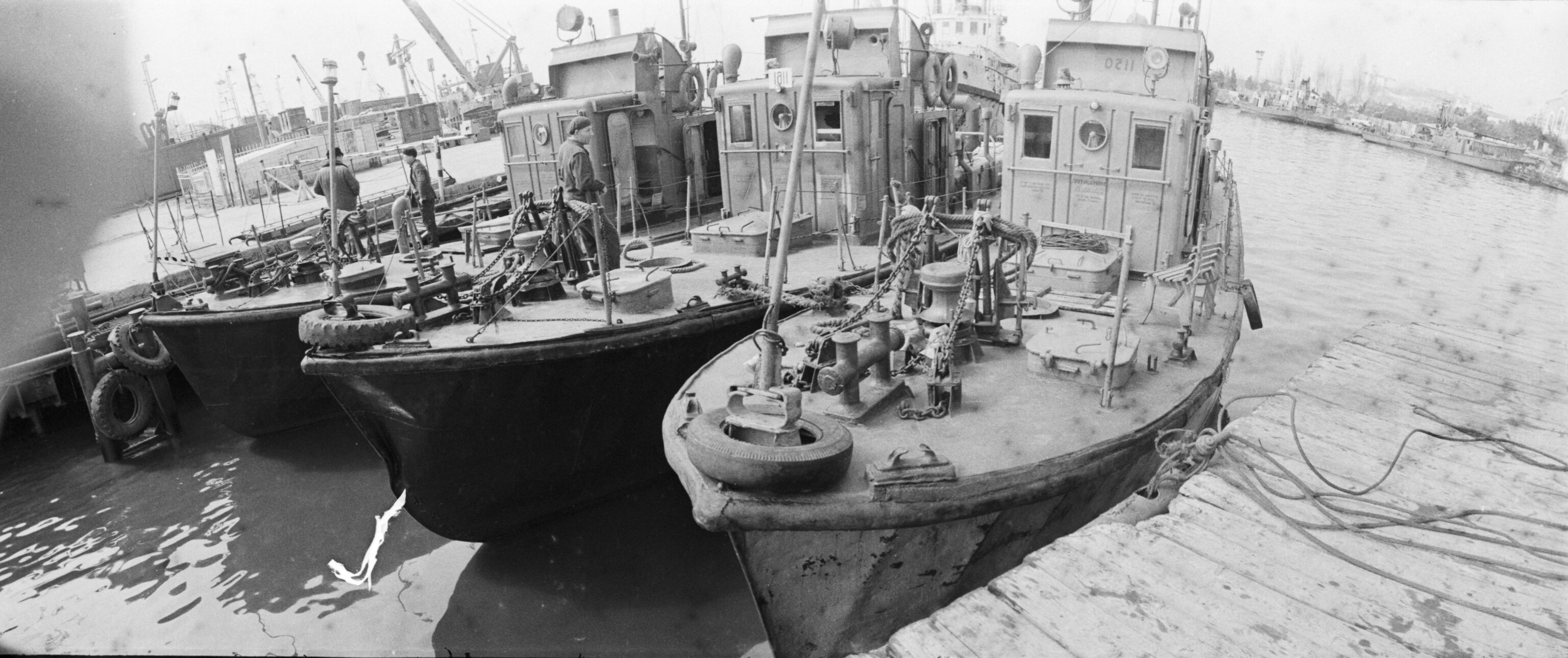This captivating black-and-white photograph reveals a dock bustling with maritime activity, showcasing three side-by-side fishing boats or working vessels made of what appears to be steel, nestled tightly against each other in calm waters. The photo is angled, not taken straight on, providing a dynamic perspective of the scene. The boats, similar in design, feature rectangular pilot houses with an additional structure rising above them, and are adorned with various hardware and equipment. The boat on the far right has a gray, weathered hull, while the two on the left have dark black hulls.

Each vessel is equipped with spare tires and metal devices for securing lines, indicative of their utilitarian purpose. The middle boat has a man on the top deck looking to his right, while the boat on the left also has men on top, seemingly engaged in conversation or work. The dock on the right is wooden, strewn with ropes and chains, and runs parallel to the boats, facilitating their mooring.

In the backdrop, across the water, a sprawling city shoreline dotted with larger vessels and infrastructure is visible, including a prominent crane and various buildings, hinting at a larger harbor or industrial area. The aged, rectangular photograph itself bears signs of wear, including small gray spots and a noticeable white scratch off the bow of the middle boat. The sky looms gray and indistinct, adding to the timeless, almost melancholic ambiance of this maritime tableau.